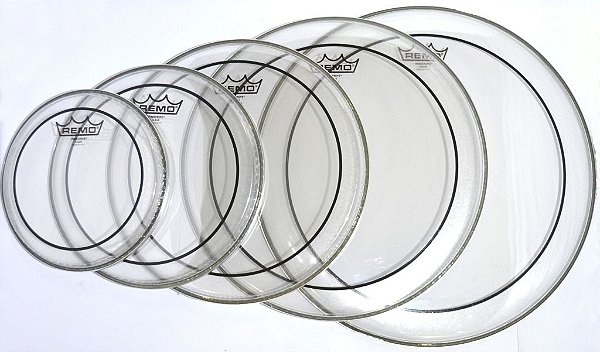The image features five translucent, circular plates arranged in a row from left to right, gradually increasing in size and diameter. The smallest plate is on the left, and the size progression creates an almost optical illusion due to their transparency. Each plate bears a black circular sticker with the brand name "REMO" in bold capital letters, accompanied by an illustration of a four-pointed crown above the text. The background of the image is white, accentuating the clear nature of the plates, as only their outlines are prominently visible. The simplicity of the color scheme, primarily whites and blacks, draws attention to the objects' minimalist design and the distinct arrangement, which appears centered horizontally within the frame.